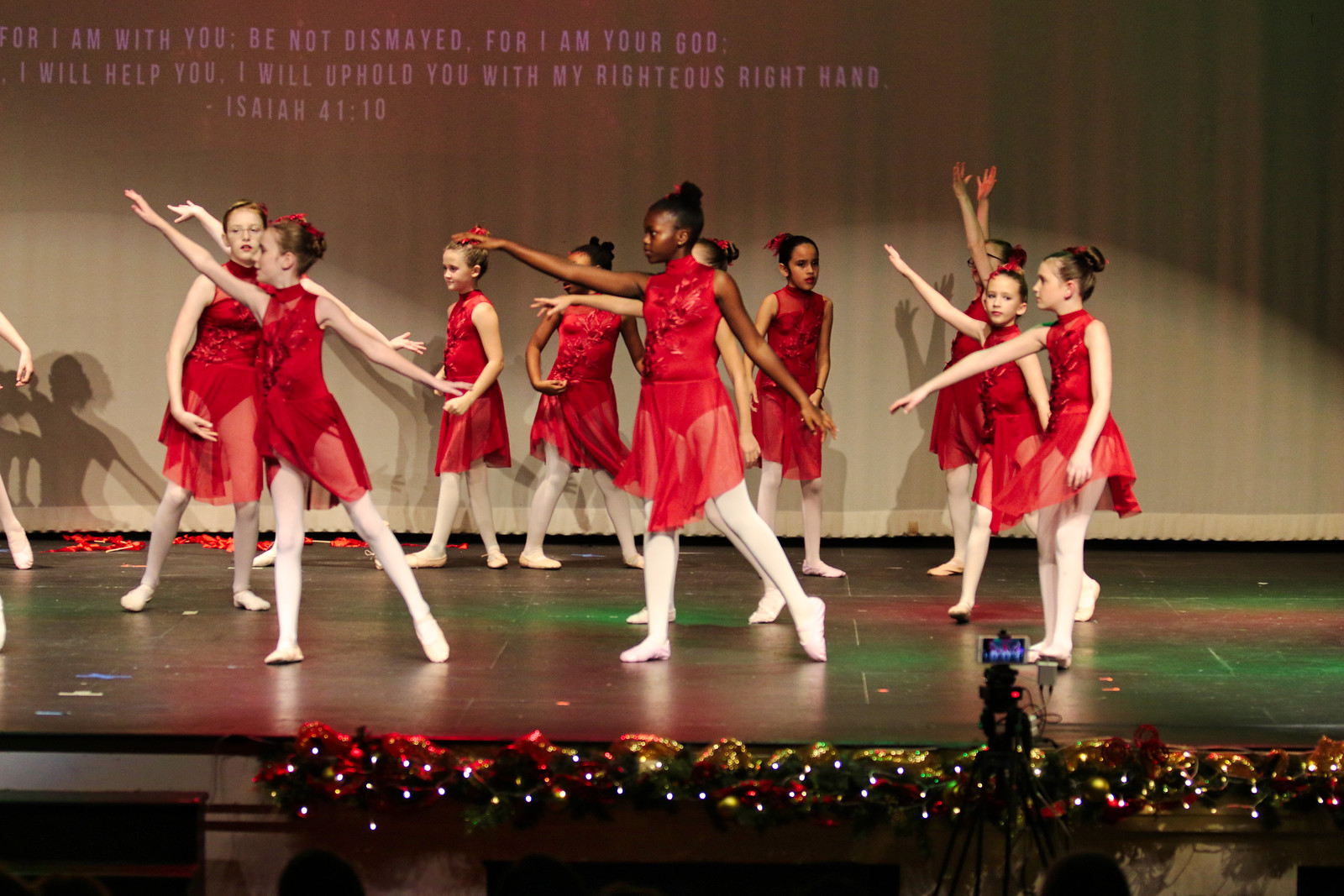This image captures an indoor scene at what appears to be a Christmas recital or concert, likely held in a theater or school auditorium. The stage is adorned with Christmas decorations along the bottom edge, including white lights, gold bells, ornaments, wreaths, and possibly gold tinsel. The stage itself seems to be dark brown or black, illuminated by spotlights and accented with green and red lights.

On stage, a group of girls of varied ethnic backgrounds—both Caucasian and African American—are performing. They are all dressed uniformly in vibrant red dresses that reach up to their necks and feature short sleeves and sheer, flowy skirts. Beneath the skirts, they wear red or white undergarments, complemented by white tights and ballerina slippers. Their hair is uniformly styled in buns.

The girls are striking a poised dance pose, with their right arms extended upward diagonally to the left, and their left arms pointing downward diagonally to the right. In the front right corner of the stage, Christmas lights add to the festive atmosphere. Behind the performers, a white sheet serves as a backdrop, onto which an inspirational message from Isaiah 41:10 is projected in pink text: "For I am with you, be not dismayed, for I am your God. I will help you, I will uphold you with my righteous right hand."